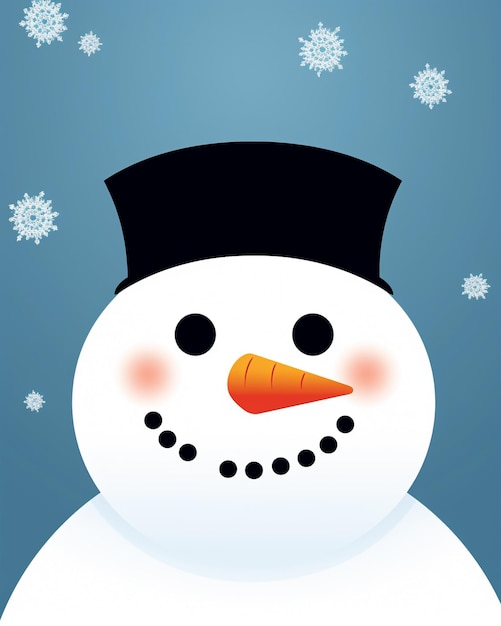This image showcases a computer-generated snowman against a wintry, grayish-blue background. The cheerful snowman features a slightly oval head adorned with two black circles for eyes and a smiling mouth made up of several black dots—though one dot appears to be missing, giving it a slightly imperfect charm. A prominent carrot nose and rosy red cheeks add to the festive feel. Completing his ensemble is a black hat, about half the height of a typical top hat. Below the head, the top portion of his body is visible, with no third layer depicted. The background is filled with intricately detailed snowflakes of varying sizes, enhancing the wintery atmosphere. The detailed craftsmanship of the snowflakes suggests the image could be the cover of a Christmas card or postcard, capturing the essence of a joyful winter day.